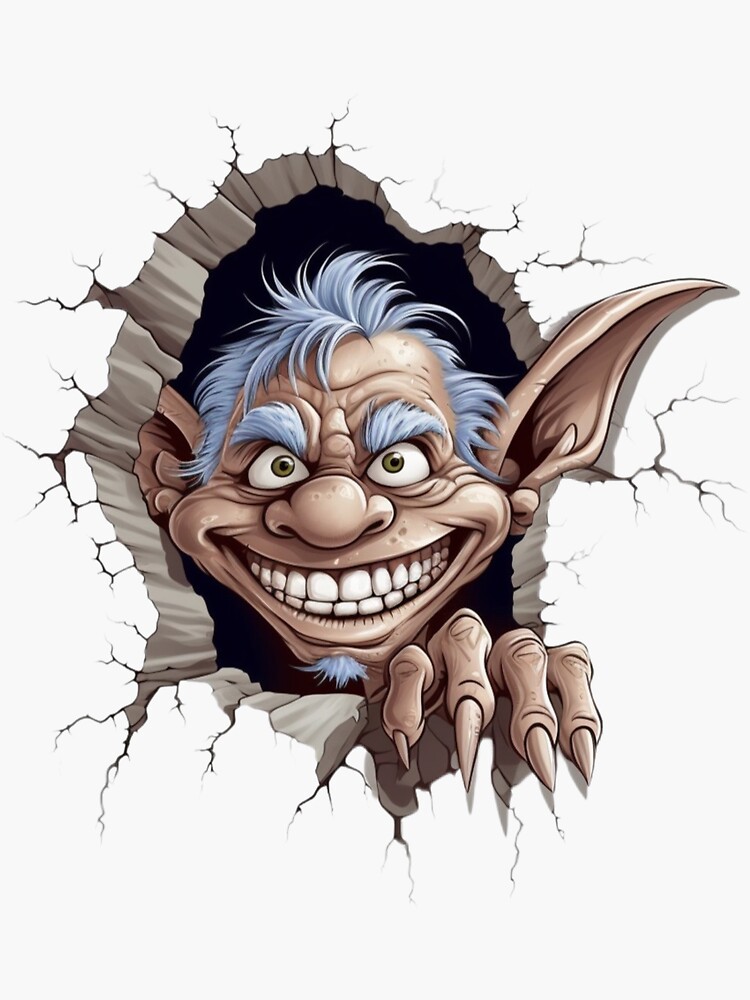In this cartoon-style image, we see a digitally created goblin or troll character emerging from a jagged, cracked hole in a primarily white wall. The hole, with its irregular, jagged edges, resembles a break caused by a forceful impact. Peering out from this hole is the goblin's face, viewed directly from the front.

The goblin's head features an evil, devilish grin showcasing its white teeth. It has two white eyes with green pupils, and a wrinkled, bulbous nose with visible nostrils. Tufts of light blue hair and bushy blue eyebrows, along with a noticeable soul patch, frame its face. The right-hand side of the goblin reveals one pointed ear sticking out, while the left ear remains partially tucked underneath. Resting on the edge of the hole is the goblin’s left hand, prominently displaying long, sharp, menacing nails. The goblin’s skin is light brown-tan, contributing to its overall eerie and menacing appearance.